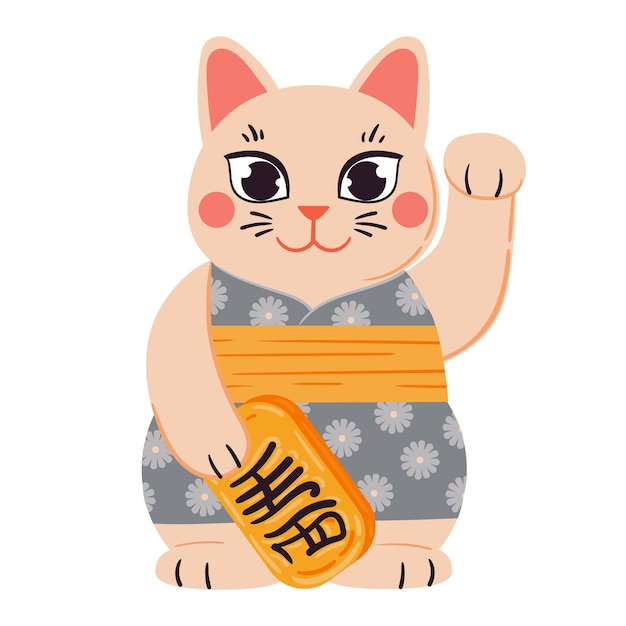This is a detailed digital illustration of a traditionally-styled lucky cat, often seen in shops to attract fortune. The lucky cat, rendered in a peachy beige tone, stands against an all-white background, smiling warmly at the viewer. It features salmon-colored insides of the ears and soft pink blush circles on its cheeks. The eyes are large and expressive, surrounded by black outlines including black eyebrows and whiskers.

The cat is adorned in a sleeveless, traditional Chinese-inspired dress that predominantly features shades of gray with intricate gray flower patterns. An orange band accentuates the midsection, adding contrast to the outfit. One arm is raised, extending a gesture of welcome, while the other holds a golden plaque inscribed with Chinese characters in black. The cat's hands and feet exhibit black lines, suggesting either claws or spaces between toes and fingers.

This meticulously crafted illustration, executed in Photoshop, captures the charm and cultural significance of the porcelain lucky cat sculptures commonly displayed in restaurants and shops to bring prosperity and wealth.